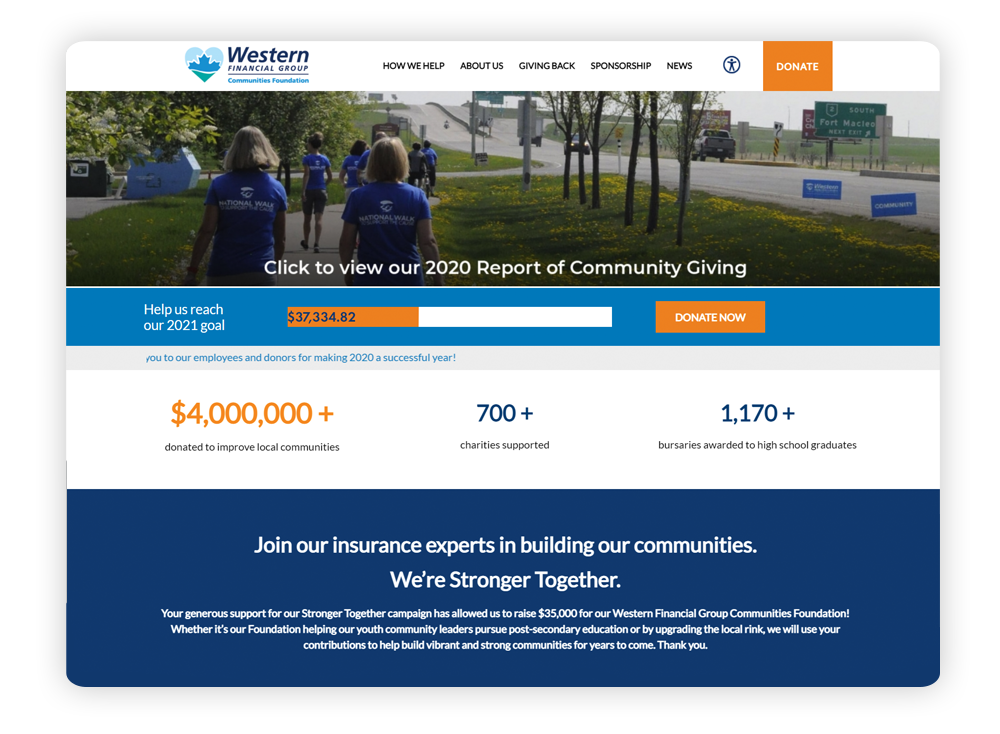Capturing the essence of the Western Financial Group Communities Foundation's website, the homepage presents a cohesive blue, white, and green color scheme. The branding at the top prominently displays the "Western Financial Group Community Foundation" name, with "Community Foundation" in a lighter blue and smaller font, and "Western Financial Group" in a darker blue. Adjacent to the text is a distinctive logo featuring a heart with a blue upper segment and a green lower segment, with a leaf in the center.

Navigation options arrayed at the top of the page include "How We Help," "About Us," "Giving Back," "Sponsorship," "News," and a "Donate" button. Central to the page is a photograph depicting approximately six individuals walking on a sidewalk next to a road, all sporting matching blue t-shirts emblazoned with "National Walk" and the Community Foundation’s logo.

Below the image, notices encourage viewers to "Click to view our 2020 report of community giving," and to "Help us reach our 2021 goal." There is a real-time update of funds raised, alongside another donation prompt.

Further down, the site celebrates its achievements: $4 million donated to improve local communities, support extended to over 700 charities, and 1170+ bursaries awarded to high school graduates. A call to action invites visitors to join the insurance experts in community-building efforts, highlighting the successful fundraising of $35,000 for the "Stronger Together" campaign. The text expresses gratitude for contributions that aid youth community leaders' education and local community enhancements, emphasizing the long-term commitment to fostering vibrant and strong communities.